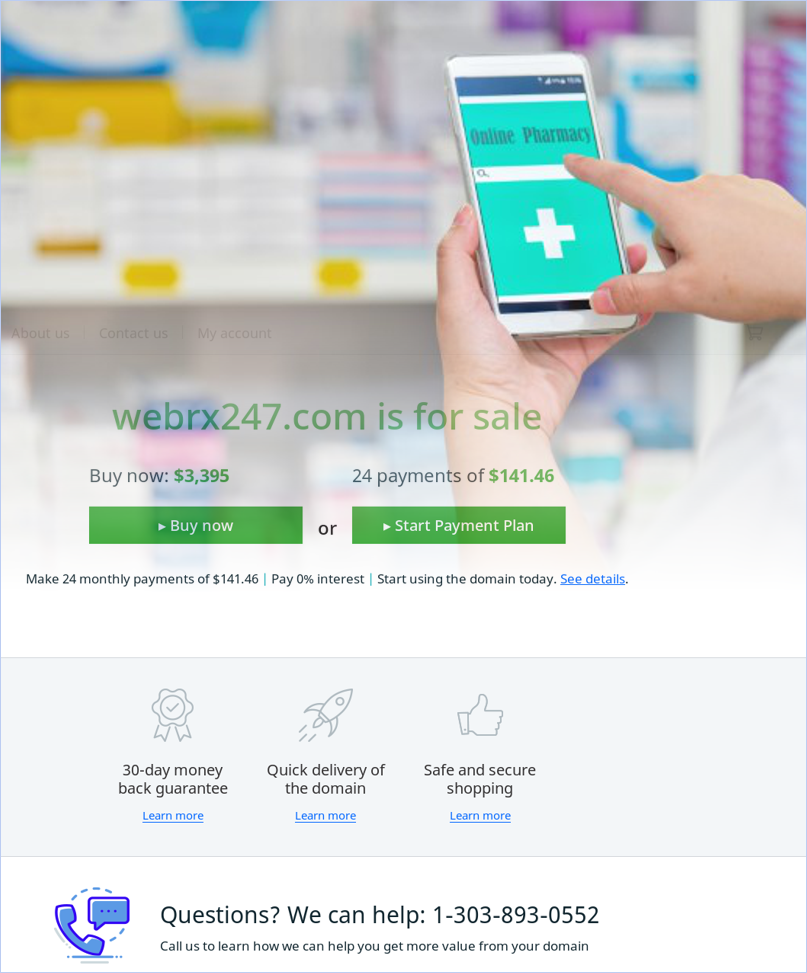A highly polished, computer-enhanced advertisement showcases a vibrant, full-color portrait image. The composition predominantly features two hands of a white woman, with polished nails, delicately holding a smartphone. The woman's finger points at the screen, which prominently displays an online pharmacy logo with a cross symbol. The backdrop is a blurred scene inside a pharmacy, easily identifiable by the vaguely discernible shapes, sizes, and colors of various prescription drug bottles lining the shelves.

The lower 40% of the image contains textual information about the domain "webrx247.com" being available for purchase. It details the buying process, offering the domain for a lump sum of $3,395 or a payment plan of 24 monthly installments at $141.46 each, with no interest. The ad encourages immediate start of domain usage upon purchase. For inquiries, viewers are directed to contact the provided help number.